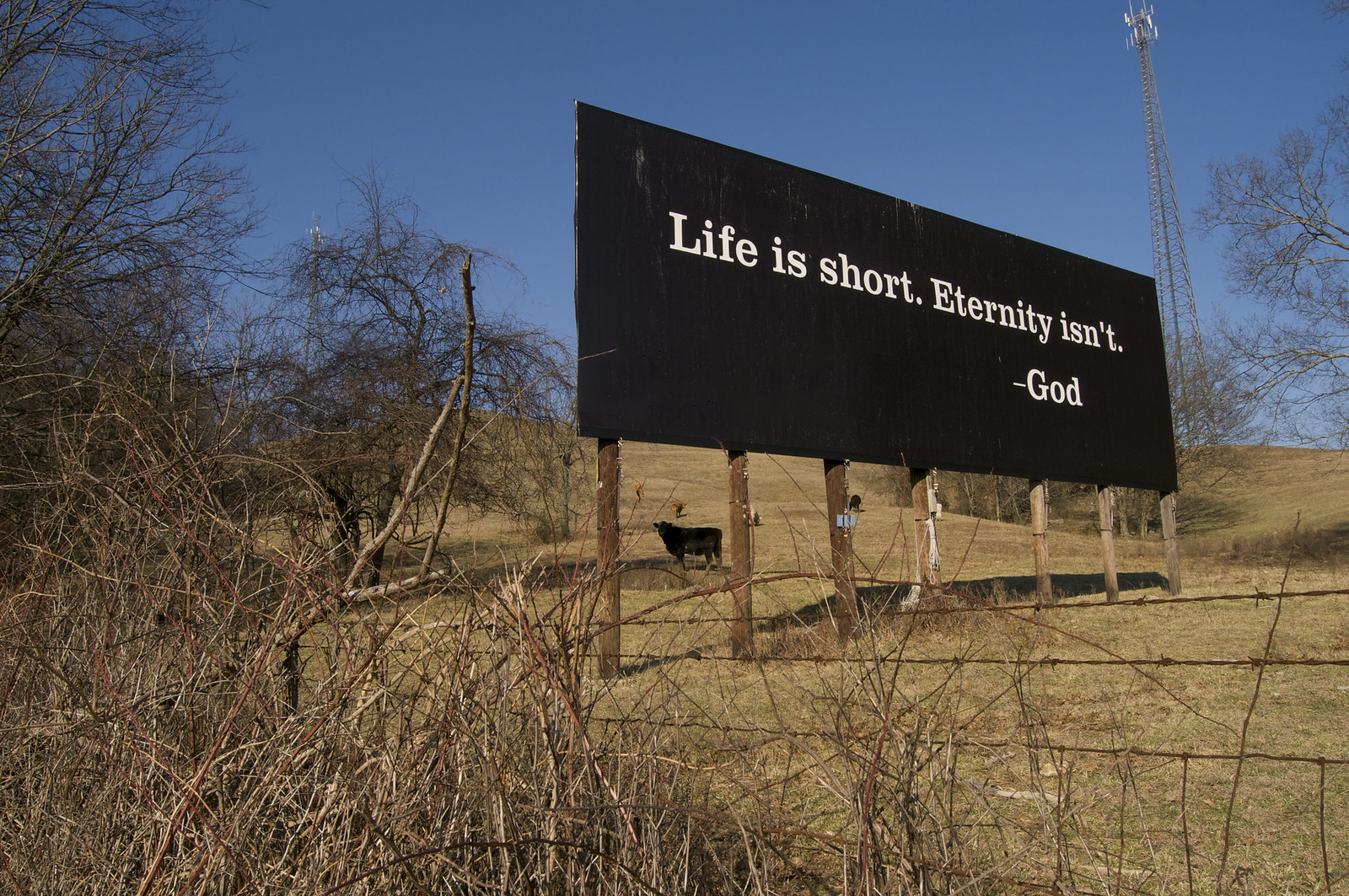This photograph captures a rural pasture under clear blue skies, dominated by a large black billboard with white text that reads, "Life is short, Eternity isn't - God." The billboard, which stands on wooden posts, is surrounded by barren trees, tree branches, and a barbed wire fence that marks the boundary of the pasture. The grassy area is primarily brown with sparse patches of green, indicating a dry and arid environment. In the background, several cows can be seen, including a notable black cow positioned directly behind the billboard. Additionally, a lattice-type tower, possibly a cell or radio tower, is visible to the right of the billboard on a hill, with another similar structure further up the hill to the left. This setting highlights the juxtaposition of modern elements like the cell tower with the timeless message on the billboard, all within a serene yet stark rural backdrop.